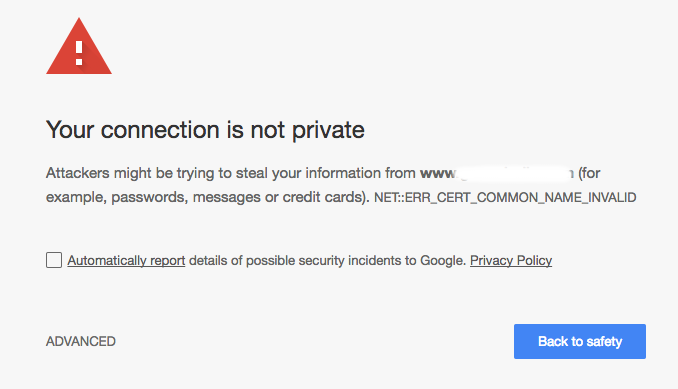This image captures a screenshot displaying a security warning message from a web browser. In the upper left corner, there is an exclamation mark inside a red triangle, indicating an alert. Below this symbol, the text reads "Your connection is not private," warning that attackers might be attempting to steal information from the website (with the URL partially obscured). It specifies that sensitive information such as passwords, messages, or credit card details could be at risk. The error specified is "NET::ERR_CERT_COMMON_NAME_INVALID."

Directly beneath this warning, there is an option to automatically report details of possible security incidents to Google, accompanied by a link to the privacy policy. In the lower left corner, users are presented with the option to access "Advanced" settings, while in the lower right corner, there is a blue rectangular button labeled "Back to safety" that users can click to exit the unsafe connection.

The entire screenshot is within a rectangular frame, with a background color of light grey.